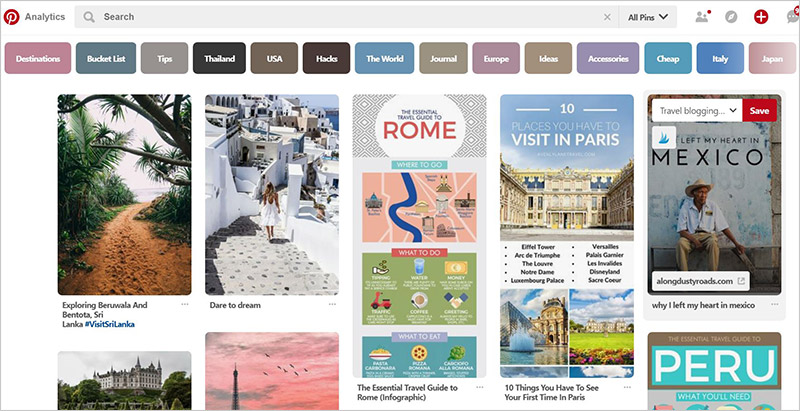This image is a screenshot of a Pinterest app interface. In the upper left-hand corner, the Pinterest logo is clearly visible, affirming the app’s identity. To the right of the logo, there is a prominent search bar, inviting users to enter their desired queries. Beneath the search bar, there is a row of approximately 15 tags, which users can utilize to refine their search results according to specific categories or interests. The main section of the screen showcases a variety of tiled pictures, each representing different vacation destinations. Noteworthy among these images are scenic views of Santorini, Greece; iconic landmarks in Rome, Italy and Paris, France; as well as vibrant snapshots of Mexico. It appears that the user has specifically filtered their search results to focus on vacation spots, resulting in a visually appealing and diverse collection of travel-related content.